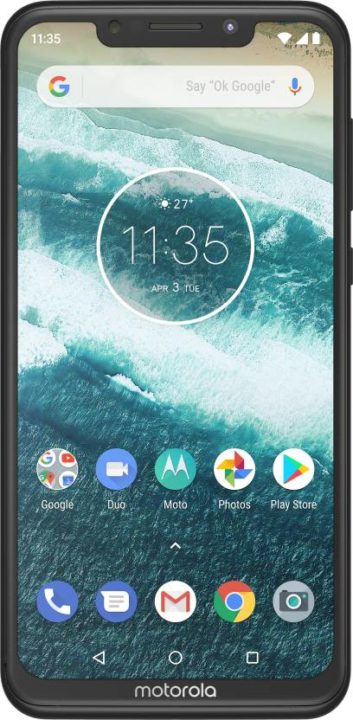The image showcases the front screen of a Motorola smartphone, which is turned on and displaying various features. At the top of the screen is a Google search bar, allowing for quick access to internet searches. Below the search bar, in the center of the screen, there's a circular widget providing the current weather, time, and date, offering convenient at-a-glance information. 

Further down, there are two rows of widgets. The first row includes a folder for Google apps, Duo, Moto, Photos, and the Play Store. The second row features a phone icon on a blue background with a white phone graphic, a messaging icon also on a blue background with a white text bubble, a Gmail icon marked by its recognizable red and white envelope on a white background, the Chrome browser icon depicted as a circle with green, red, and yellow segments around a blue center, and finally, a camera icon set on a gray background.